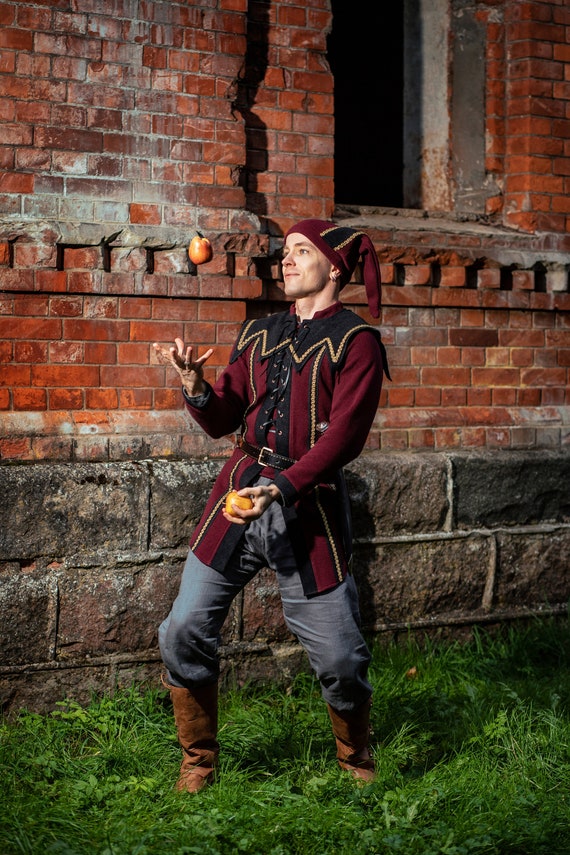The photograph captures a man in an elaborate jester costume, juggling apples while standing in long green grass. Behind him looms a cobblestone and brick building, reminiscent of an old castle or renaissance fair backdrop. The structure features dark gray, rectangular stones at its base with reddish-brown bricks above, interspersed with a shadowy, clouded window. The jester, adorned in a maroon hat with dangling ends and a matching maroon jacket with a detailed black collar, sports gray pants, a black belt, and knee-high brown boots. He has one apple held aloft in mid-air while grasping another in his hand, indicating the motion of juggling.